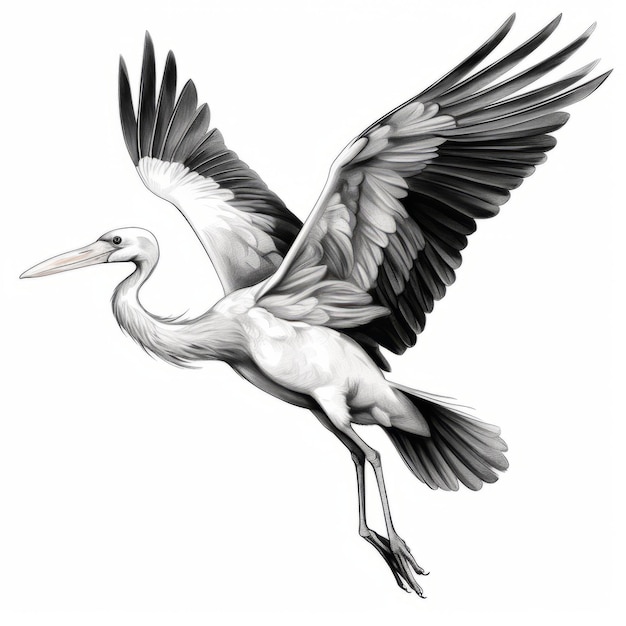The image depicts an intricately detailed pen and ink drawing of a large bird in flight, possibly a crane or stork, characterized by its elongated neck, long legs, and expansive wingspan. The bird, rendered predominantly in black, white, and gray shades, features a slightly pinkish or orangish beak. It has a graceful, curved neck adorned with feathers underneath and a smooth, predominantly white body. The beady eye is focused forward, indicative of its mid-flight or takeoff stance.

The wings are extended wide with distinct visual contrasts: the leading edges of the wings are white, transitioning to contour feathers that are lightly shaded with black lines, and ending in dark, black feathers along the tips and back edges. Its tail feathers mimic this pattern, being predominantly white but marked with black lines. Additionally, the bird’s long toes and talons are noticeable. The background of the drawing is left intentionally bare, spotlighting the meticulous detail and artistic finesse of the bird itself.